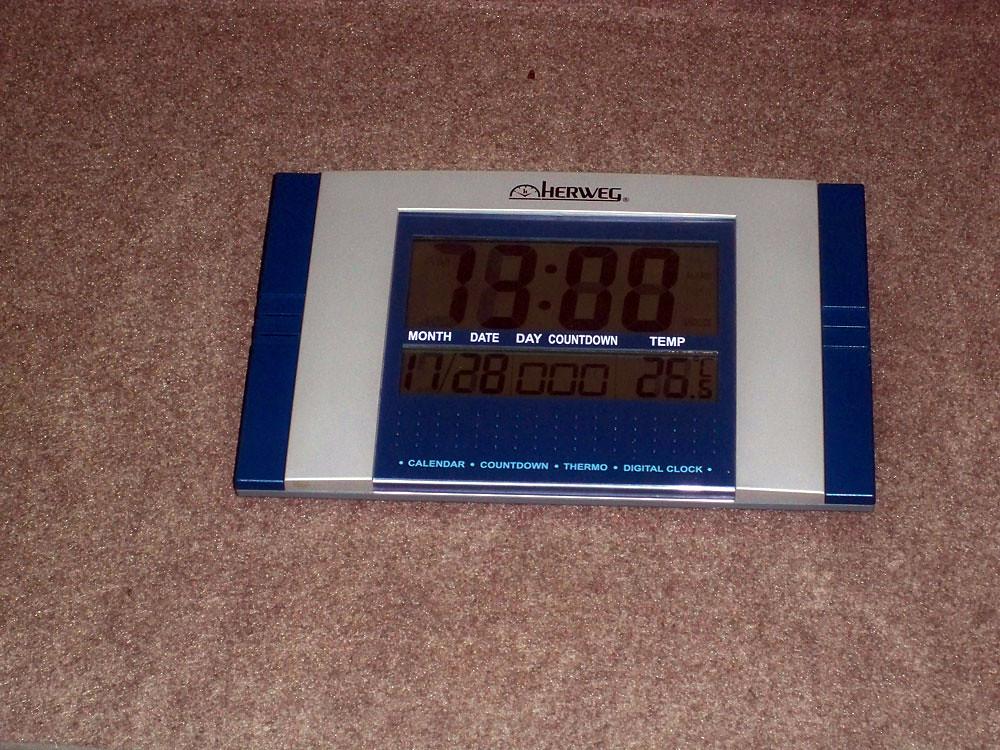The photograph captures a detailed, close-up image of a rectangular digital clock with multiple features. The clock is labeled "HERWEG" at the top and is encased in a predominantly silver or white housing with metallic blue vertical bars on either side. The clock's LCD screen displays information including the month, day, date, countdown, and temperature. Below the screen, in white and light blue text, it lists additional features such as "calendar, countdown, thermo, digital clock." The clock is placed atop a carpeted floor with a whitish, reddish hue. There are no other elements, people, or animals in the photograph.